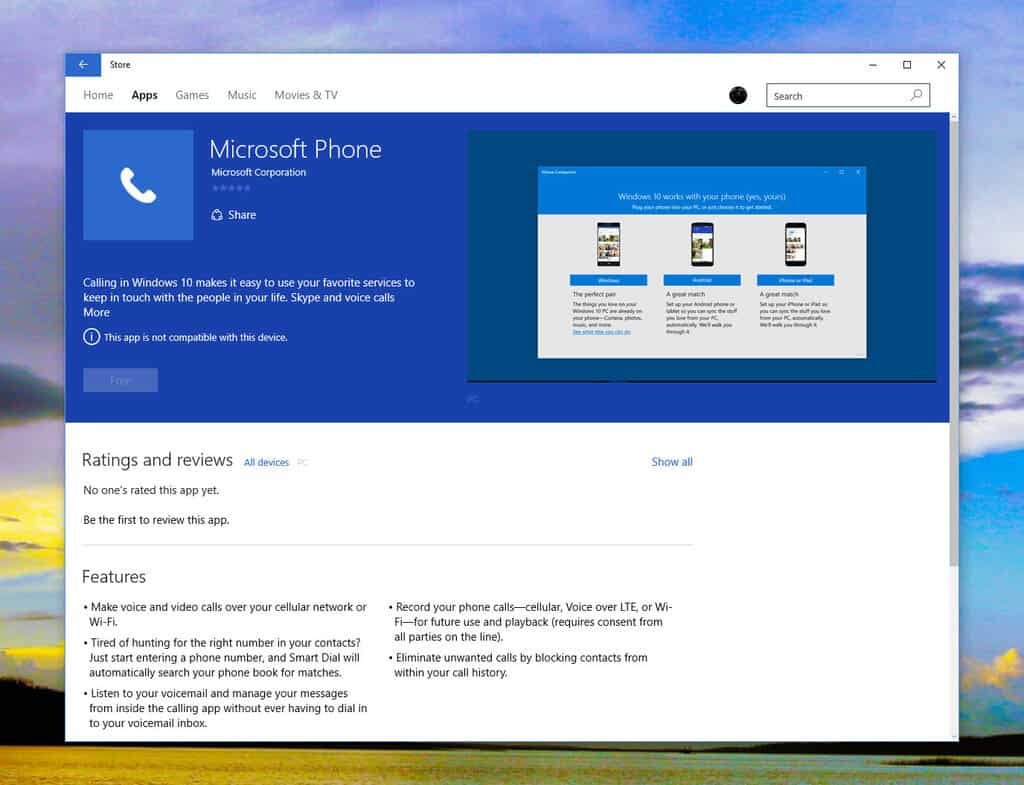This image is a detailed screenshot captured from a desktop or laptop computer. The desktop background is a picturesque scene featuring a blue sky dotted with white clouds, transitioning into a serene lake with a yellow sheen on its surface to the left. Dark, rolling hills line the horizon, adding depth to the landscape.

In the foreground, an active window titled "Store" is open, displaying the "Microsoft Phone" app by Microsoft Corporation. The app description highlights that this service enables easy communication via favorite services on Windows 10, including Skype and voice calls. However, a notice indicates that the app is not compatible with the user's current device. 

Below the app description, it is mentioned that there have been no ratings or reviews yet, inviting users to be the first to provide feedback. The app's features are elaborated upon, emphasizing capabilities such as making voice and video calls over cellular networks or Wi-Fi, Smart Dial for effortlessly finding contacts, managing voicemail directly within the app, and recording phone calls over LTE or Wi-Fi. The interface includes navigation options along the top for Home, Apps, Games, Music, Movies, and TV, with a search bar situated on the right.